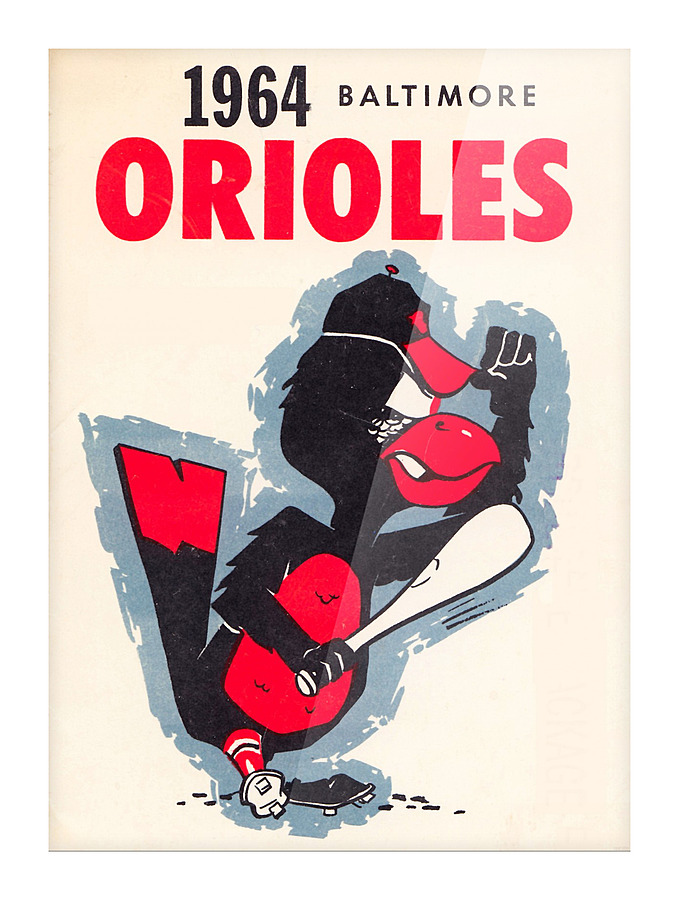This detailed image captures a vintage 1964 Baltimore Orioles advertisement. It features a cartoon bird, presumably an Oriole, which has striking black feathers paired with a red stomach, beak, and tail. The bird is depicted wearing a black and red cap, red socks, and looks quite serious as it holds a baseball bat in one hand while adjusting its cap with the other. A subtle blue outline enhances the character's presence against the aged, off-white background of the piece. The text is minimalistic yet bold, with "1964 Baltimore" rendered in black and "Orioles" in red, echoing the bird's vibrant colors. The poster appears to be screen-printed and has a distinctly aged, yellowing appearance, fitting for something from the 1960s, and exudes a retro, collectible feel.